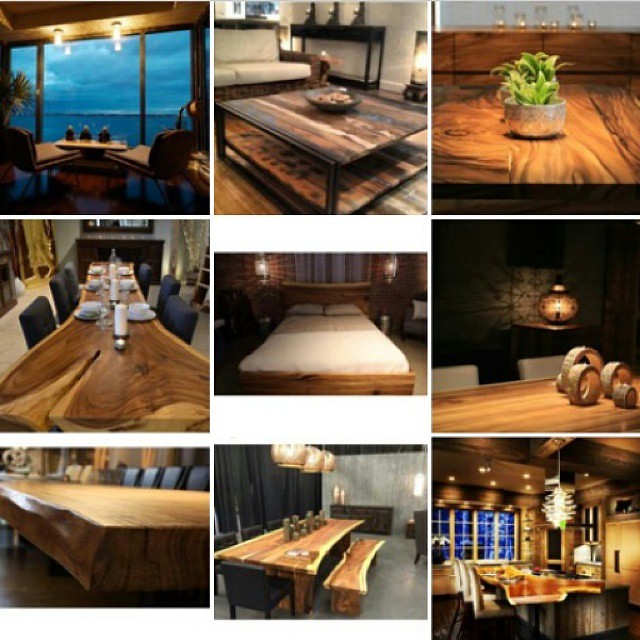A grid of nine photographs, arranged three across and three down, showcases various rooms and wooden furnishings within a house. The top left image captures an indoor balcony view with an ocean backdrop at nighttime, framed by windows, featuring a small table set with three short objects and a plant to the left, flanked by two seats. The top middle photograph displays a cozy living room with a rattan-looking couch adorned with cream-colored cushions and a wooden coffee table holding a small bowl with light brown objects. The background features a dining cabinet topped with three items and illuminated by a tall light. The top right image highlights a wood grain table with a small bowl sprouting green plants, situated in front of shelving that holds six candles in glass encasements.

The middle left photograph shows a long dining table with gray chairs, set for six with plates and bowls, and adorned with candles along the center. An artificial fireplace with a mirror or picture tops the scene. Centered in the middle row, a queen-size bed with clean white sheets is set in a brown bed frame, representing the master bedroom. The middle right photo captures a table with two cream-colored chairs, featuring circular objects in the middle and an oval light fixture in the background.

The bottom left image portrays a long brown wooden table surrounded by chairs on one side, captured from a bottom left angle. The bottom middle photo shows another long wood grain table with benches, adorned with several objects in the middle and gray walls with cabinetry at the far end. The bottom right picture presents a formal dining setting with a wooden table under a chandelier, windows in the background, and a hint of blue visible through them.